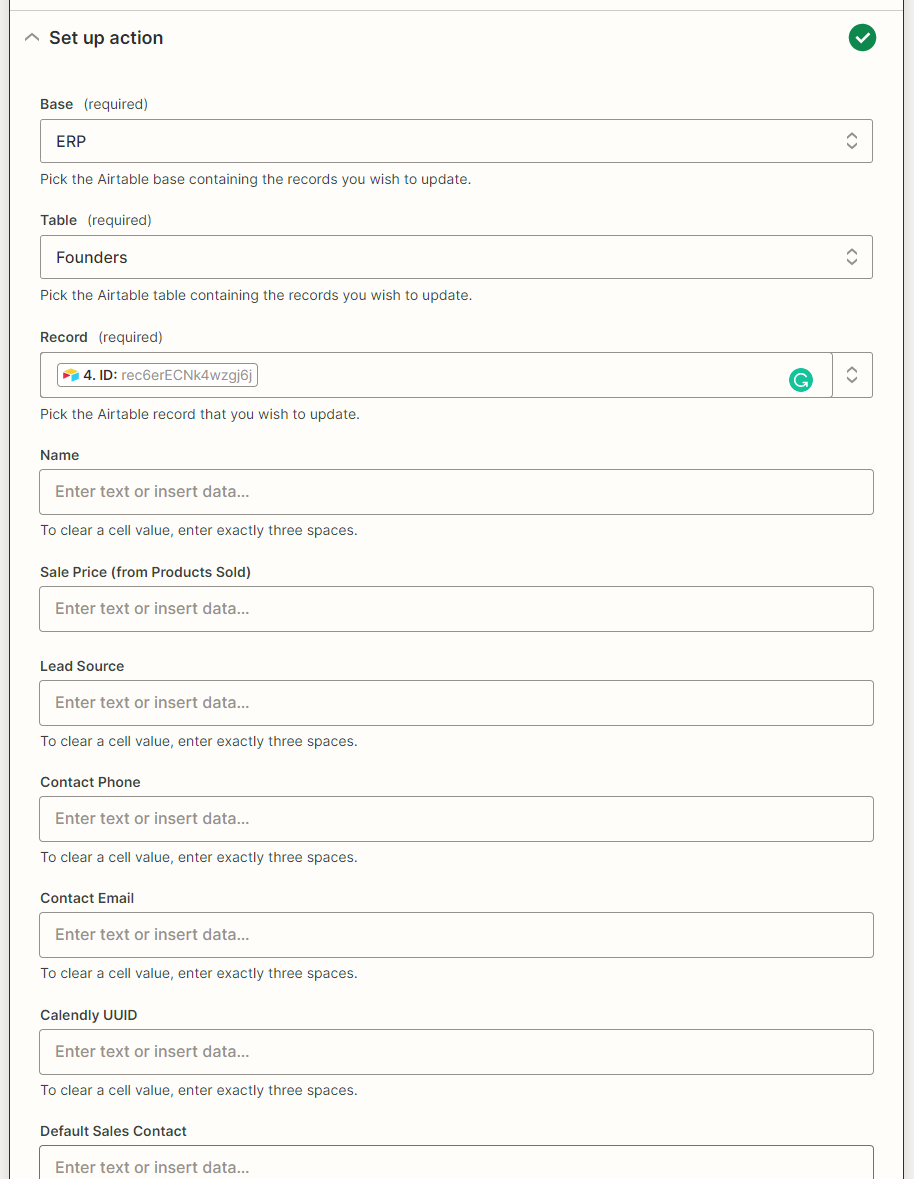The image depicts a section of a form on a website designed for setting up actions in an application. The form is bordered with thin lines on both sides and a thinner line at the top. Below the top line, there is a dark print label reading "Setup Action," accompanied by an upward arrow.

On the right side of the header, there is a round green circle with a white checkmark inside it. The form appears to be divided into sections, with each section containing fields and instructions for data input.

The first section is labeled "Base (Required)" with a drop-down menu displaying "ERP" in uppercase letters. Beneath this, an instruction reads, "Pick the Airtable Base containing the records you wish to update."

The next section is labeled "Table (Required)" with a drop-down menu showing the option "Founders." This is followed by the instruction, "Pick the Airtable containing the records you wish to update."

Further down, there is a field labeled "Required," featuring a box with a value formatted as "4-period ID: rec6eRNK4wzgJ6J." This section instructs, "Pick the Airtable record that you wish to update."

Following this, there is a series of labeled fields for entering or inserting data:

- Name: Enter Text or Insert Data
- Sale Price from Product Sold: Enter Text or Insert Data
- Lead Source: Enter Text or Insert Data
- Contact Phone: Enter Text or Insert Data
- Contact Email: Enter Text or Insert Data
- Calendly UUID: Enter Text or Insert Data
- Default Sales Contact: Enter Text or Insert Data

Each label is paired with the instruction to "Enter Text or Insert Data," emphasizing the requirement to input specific information or select from provided data options.